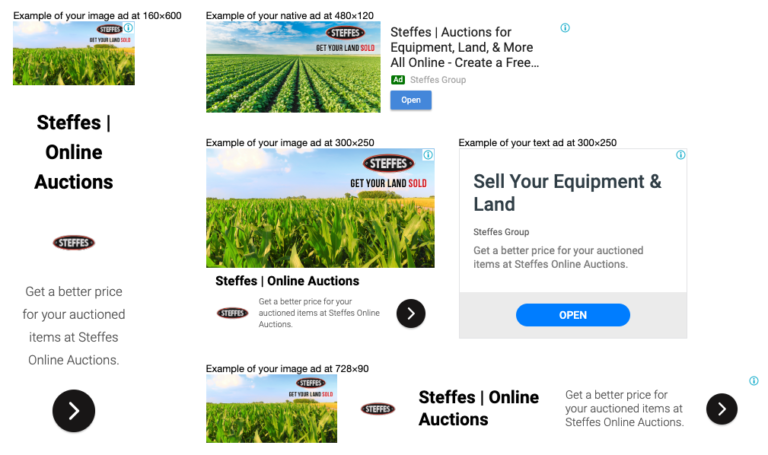This is a detailed screenshot of an online auction website, primarily promoting services for selling equipment and land. On the right-hand side of the interface, encased in a grey border, is an advertisement encouraging users to "sell your equipment and land," followed by explanatory text and a bold blue button labeled "open." This section's backdrop is white, contrasting with the blue button, which is on a blue background set against another grey layer.

Centrally displayed are three vivid images of what appear to be cornfields or similar agricultural landscapes, with another field image positioned at the top left corner. Each of these pictures is prominently branded with an oval-shaped logo featuring "STEFs" in white text on a black background, accompanied by the slogan "get your land sold." None of the images have borders, seamlessly blending into the website’s clean, white background.

On the bottom part of the screenshot, there's a right-pointing arrow set against a black background, possibly indicating navigation controls. The right-hand side and parts of the bottom are filled with white space, maintaining a minimalist aesthetic.

Additionally, the bottom right corner of the screenshot includes the text "STEFs online auction" in bold, with the slogan "get a better price for your auctioned items at STEFs online auctions" in smaller text beneath it. Similarly, the left-hand side of the screen features identical text, ensuring that the promotional message is clearly conveyed.

The entire layout is presented in a landscape orientation, combining functionally organized sections with visual simplicity to emphasize the auction services provided by STEFs.